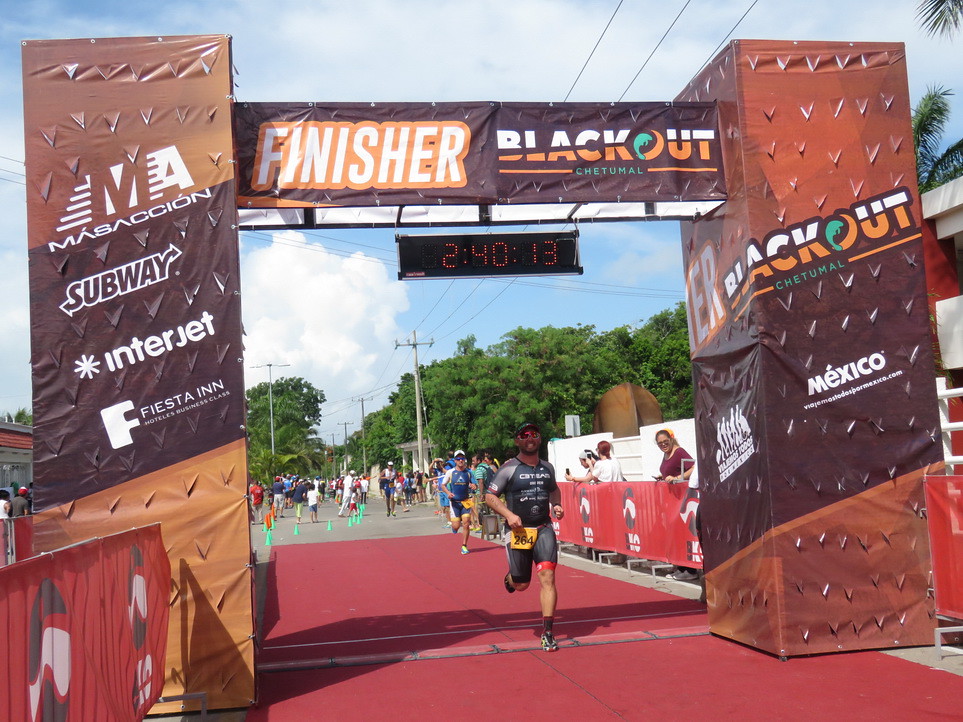The photograph captures the vibrant moment of a man crossing the finish line at a marathon on a sunny day. The scene is set against a backdrop of a bright blue sky adorned with puffy clouds and framed by both palm and green trees, indicative of a summer event. The road, lined with spectators on either side, is marked by telephone poles and wires overhead.

Central to the image is a distinctive finish line archway composed of two tall, striped rectangular pillars in shades of light brown and dark brown. Connecting these pillars is a banner featuring various sponsor logos, with the words "Finisher" in white text on an orange background on the left side, and "Blackout" in white and orange text on the right side. Below this banner, a black LED timer prominently displays the race time as 2 hours, 40 minutes, and 13 seconds.

The spotlight is on a determined runner with brown skin, adorned in a gray and black running outfit, including a hat, glasses, a gray and black shirt, black biker shorts, and a yellow participant bib numbered 264 pinned at his hip. A red carpet extends from the finish line, further accentuating the moment as he strides across the archway. In the distance, more runners are visible, approaching the finish line, adding to the dynamic and celebratory atmosphere of the marathon event.